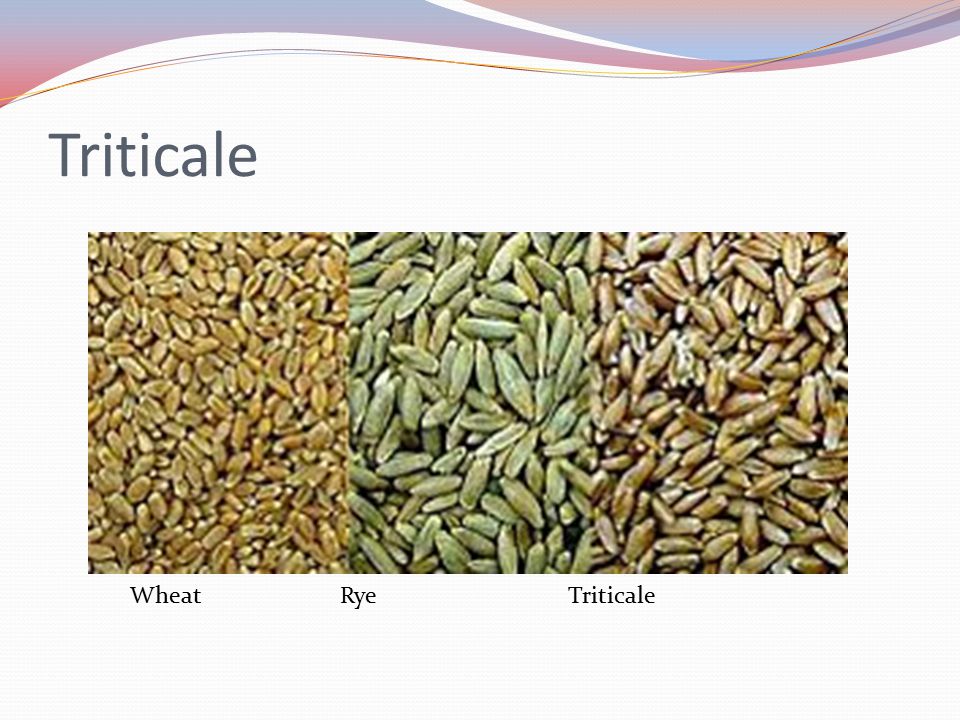The image presents a clean, white background with a stylish swoosh of pink, blue, and white gradients at the top, reminiscent of a PowerPoint presentation design. Below, bold black text in the upper left corner reads "Triticale." Centrally aligned and prominently displayed are three labeled photographs of varying grains. On the left, a yellowish grain labeled "Wheat"; in the middle, a greenish grain labeled "Rye"; and on the right, a brownish grain labeled "Triticale." Each grain is neatly contained within its respective box, making for a visually appealing and informative layout.